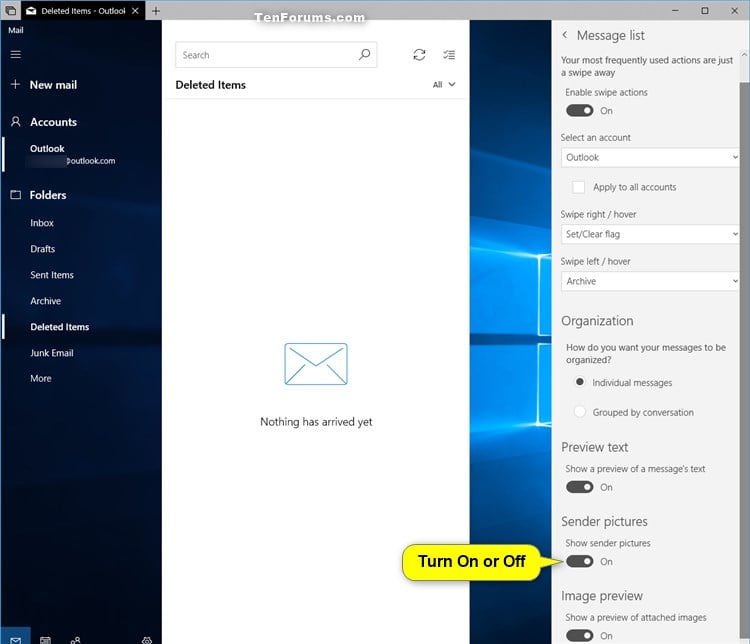This image showcases the interface of Microsoft Outlook with the focus on the "Deleted Items" folder. On the left-hand side, there is a vertical navigation menu featuring several options. At the top of this menu is the "Mail" tab. Directly beneath it is the "New Mail" option, indicated by a plus sign. Following that is the "Accounts" section, represented by a silhouette icon of a person.

Below "Accounts," the menu displays "Outlook," followed by "Folders." Within the "Folders" section, various mail folders are listed, including "Inbox," "Drafts," "Sent Items," "Archive," "Deleted Items," "Junk Email," and an option for more folders. The "Deleted Items" folder is currently selected, as indicated by its highlighted state.

To the right of the navigation menu, the main content area is divided into two sections. On the left side of this area, there is a display of the "Deleted Items" folder, which is presently empty. To the right, there is a message list section featuring toggle switches for various settings. The interface includes yellow-highlighted text indicating toggle options—one of which appears to be related to "sender pitches," currently in the on position.

The overall layout and design of the interface are consistent with the standard Outlook email client, providing users with intuitive navigation and clear organization of email folders and settings.